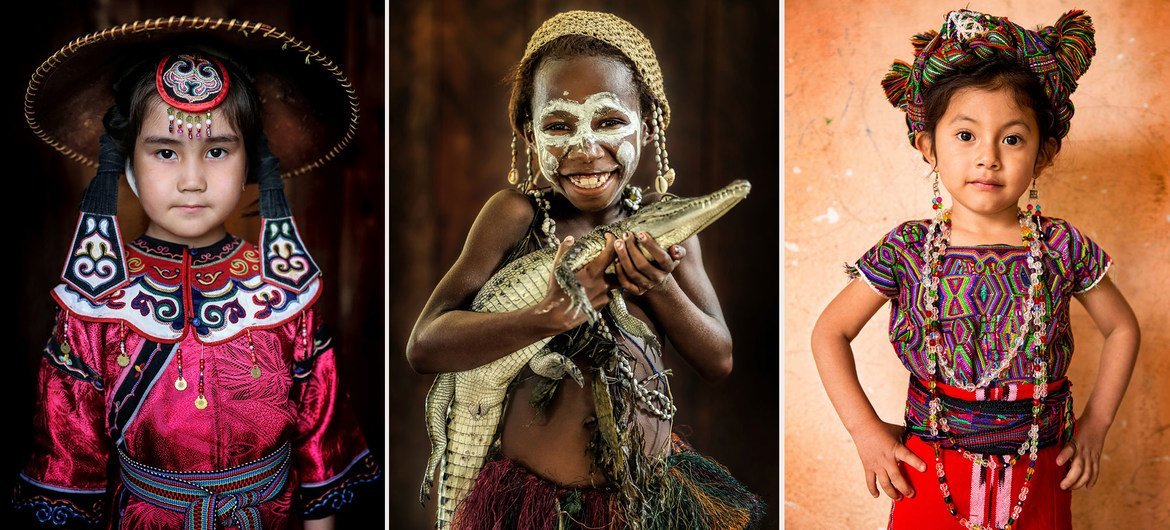In this rectangular image composed of three side-by-side photographs, each featuring a child from a distinct cultural background, the first photograph on the left shows a young girl with black hair and braids, wearing a wide-rimmed sombrero embellished with beads and a badge. She dons a red silk shirt with an ornate white collar accented in red, gold, and dark blue, along with a tied sash around her waist, evoking the attire of a traditional bullfighter. She gazes directly at the camera, exuding confidence.

The central photograph captures an African child with a beaming smile, adorned in minimal clothing. He sports a woven hat and has white face paint around his eyes and cheeks. His attire includes a colorful skirt made of tufts in red, blue, green, and yellow hues. In his hands, he gently holds a baby alligator or crocodile, which stands in stark contrast to the child's joyful demeanor.

The third photograph on the right showcases another girl, whose ethnicity remains unclear but is characterized by tan, olive skin and dark brown eyes. Her vibrant outfit consists of a multicolored shirt featuring shades of purple, gold, green, aqua, blue, and red, paired with a red skirt. She wears multiple strands of beads around her neck, and her hair is elegantly styled in a colorful bonnet. With her hands confidently resting on her hips, she similarly looks straight at the camera. The images together create a rich tapestry of cultural diversity, each child representing their heritage with pride against a neutral tan background.